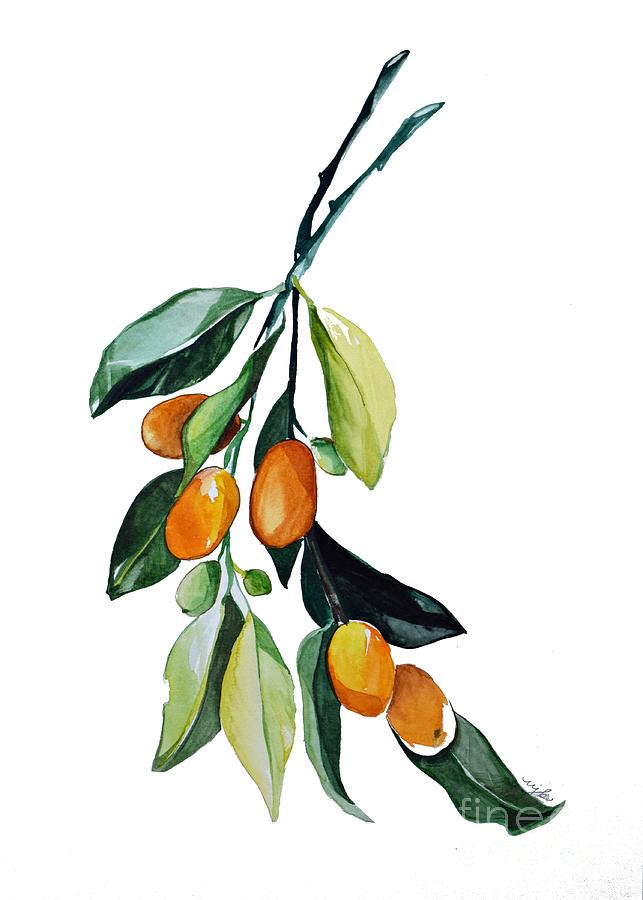This watercolor painting features a beautifully detailed depiction of two severed plant stems adorned with waxy, two-toned leaves that exhibit various shades of green, ranging from light green and yellow-green to dark green and emerald green. The artist has captured the subtle differences in the leaves, some of which are two-toned, with one half displaying a lighter or different green compared to the other. Hanging from the stems are orange, oval-shaped fruits that resemble mangoes, with five of them easily visible and three additional fruits in an unripened state. The stems and leaves converge towards the bottom of the painting, where the fruits are clustered. Set against a stark white background, the painting is subtly signed by the artist in the lower right-hand corner, with the word "fine" discernible near the signature.